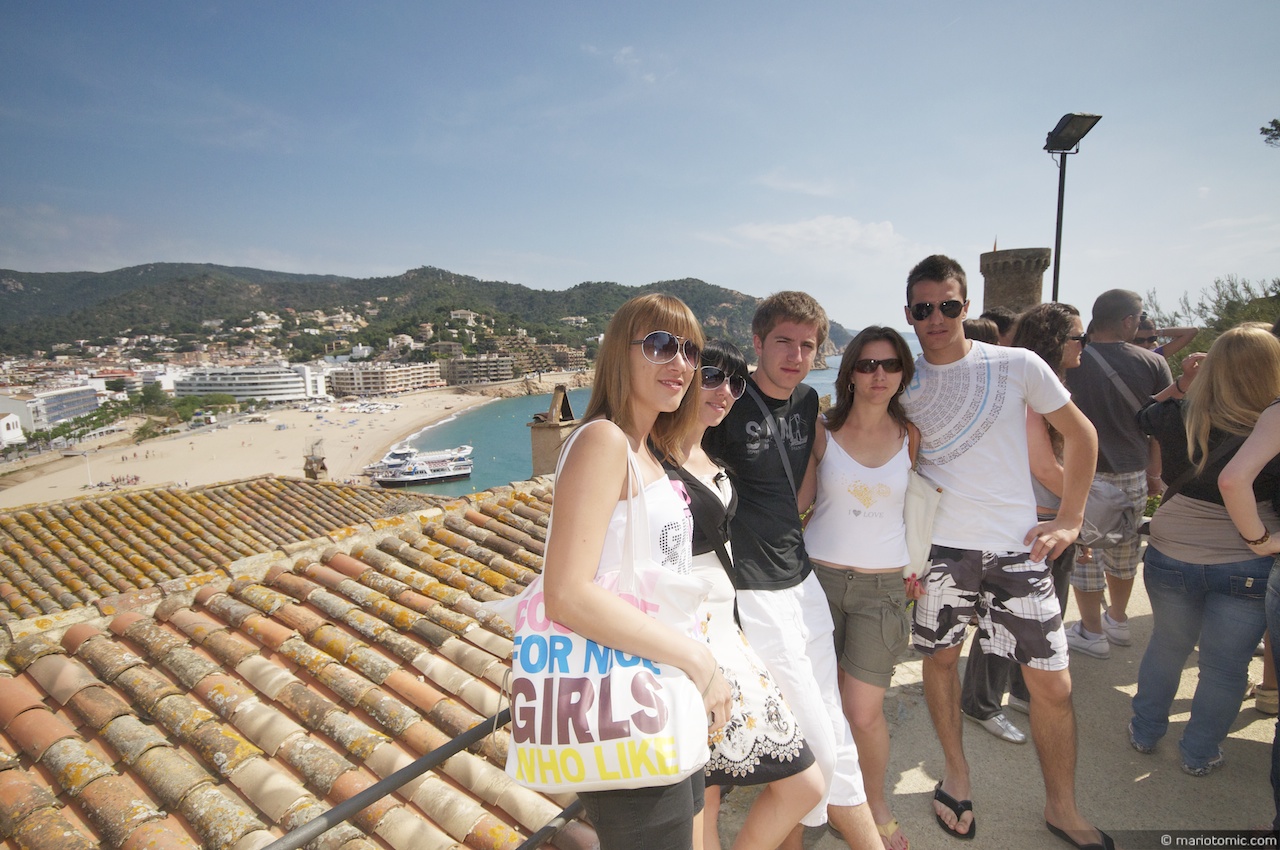A vibrant daytime photograph captures five young adults, likely in their teens or early twenties, posing joyfully for the camera amidst an outdoor coastal setting. Four of the five individuals sport sunglasses under a mostly blue, slightly clouded sky, all dressed in casual summer attire that includes shorts and flip-flops, typical of a spring break outing. The group consists of three women and two men standing on a walking space of a roof area, framed against a backdrop of a scenic coastal city. The city features numerous resort hotels and residential areas nestled along lush, green mountain ranges. The tallest woman, positioned on the far left with light brunette hair and a white blouse, holds a large bag partially obscured by her hand. To her right is a woman in a black-to-white gradient dress with black hair. The central figure is a white man with short brown hair, wearing a black t-shirt and white shorts. On his right stands a woman with brunette hair in sunglasses, a white tank top, and green shorts. The group is completed by another white man with short brown hair, donning a white t-shirt and camouflage shorts.

In the background, a white ferry or cruise ship is visible, docked at a sandy beach with bluish-green waters. Surrounding this bustling area, multiple buildings including hotels of various shapes and sizes, line the coastal city, indicating a popular tourist destination. The picturesque mountain range with dense forestry provides a majestic backdrop, enhancing the serene yet lively ambiance captured in this snapshot of a memorable vacation.